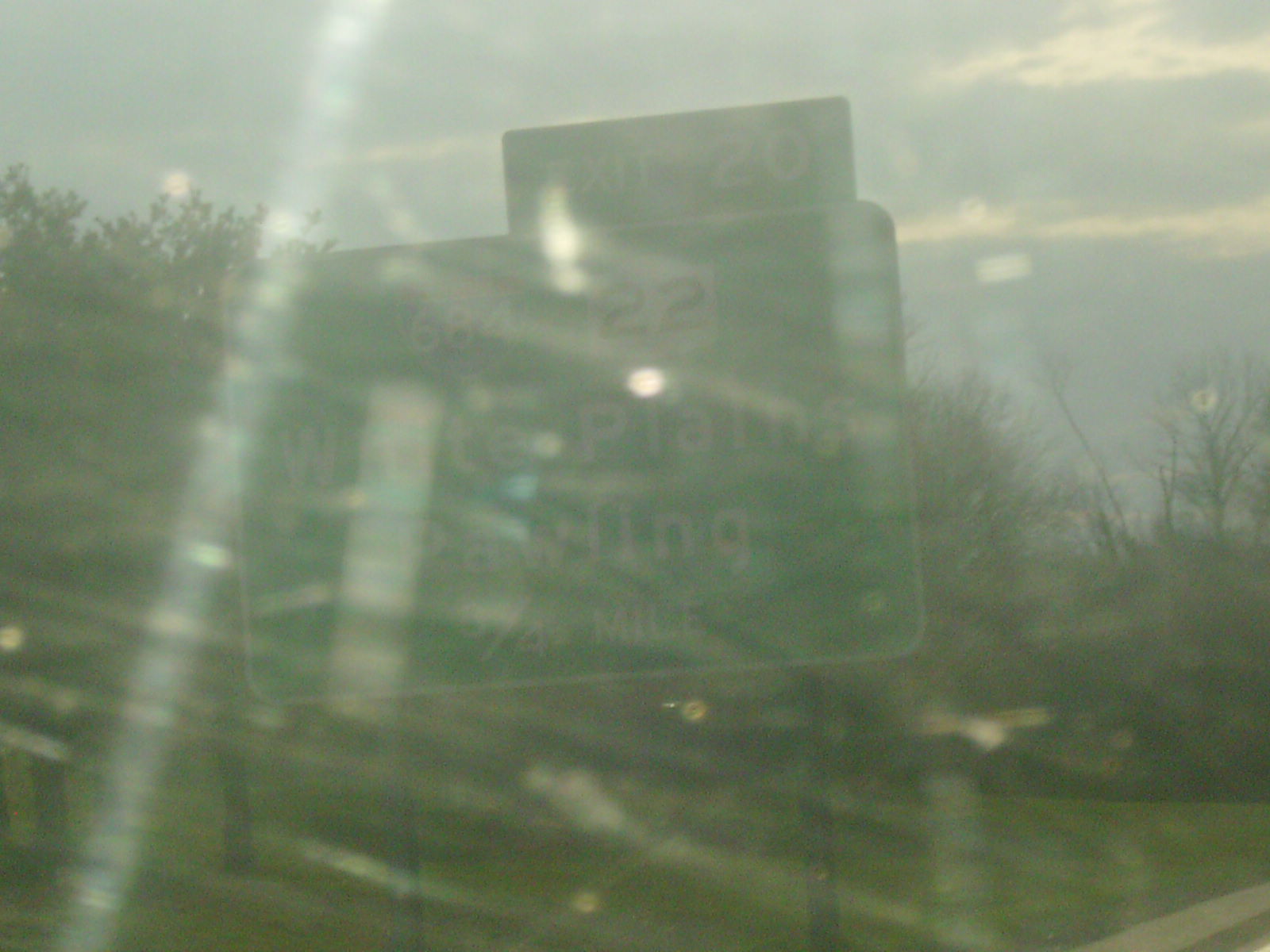A blurred, low-quality photo shot hastily from a moving car captures a scene outside the window, where a grimy layer of dirt distorts the view. Taken at high speed, the image reveals a landscape tinted with a yellowish-green hue due to the dirty window. Amidst the blur, a backdrop of trees and a blue sky scattered with white clouds is partially discernible. Prominently visible is a green road sign indicating "Exit 20" on Interstate 684, mentioning Road 22 and White Plains, with additional text suggesting a distance of three-fourths of a mile, although the poor image quality renders it nearly illegible. This snapshot clearly captures a fleeting moment on the highway, giving an impressionistic view from a car window.